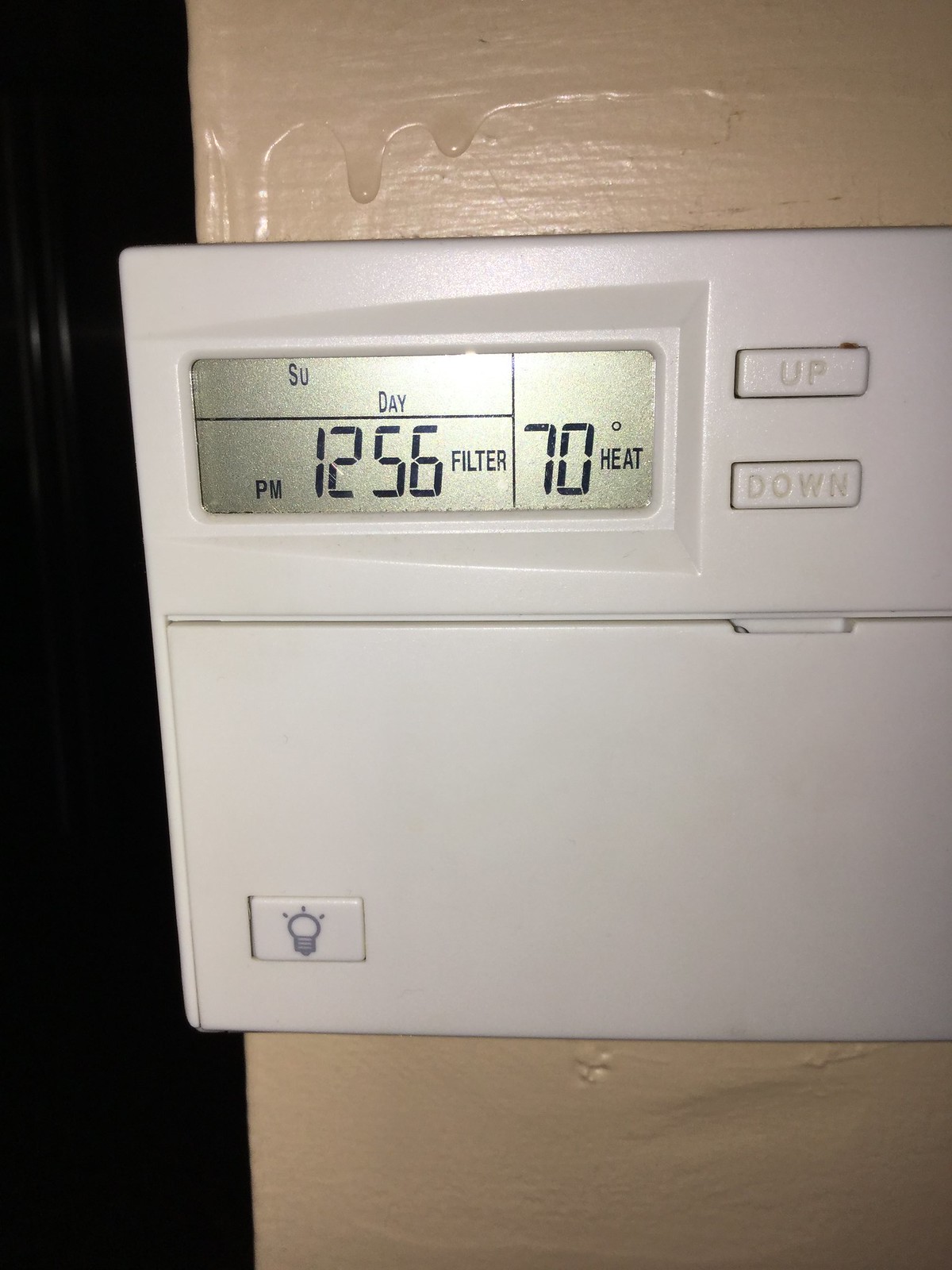A color photograph captures a close-up of a white, plasticky thermostat mounted on a poorly painted taupe wall. The image has a portrait orientation, similar to a book page, with a stark black left background likely due to a bright light shining on the thermostat, casting the surrounding area into deep shadow. The taupe wall, painted with a shiny satin or semi-gloss finish, is marred by noticeable paint drips and runs above the thermostat, and has several dings below it that were not properly spackled before painting. The thermostat itself features a small digital screen displaying "SU" (Sunday), "PM," the time "12:56," a "filter" indicator, and the temperature setting "70 degrees" in "heat" mode. Below the screen, two rectangular buttons labeled "Up" and "Down" allow for temperature adjustments. Additionally, a button with a lightbulb icon is located on the bottom left of the thermostat, presumably to illuminate the screen.